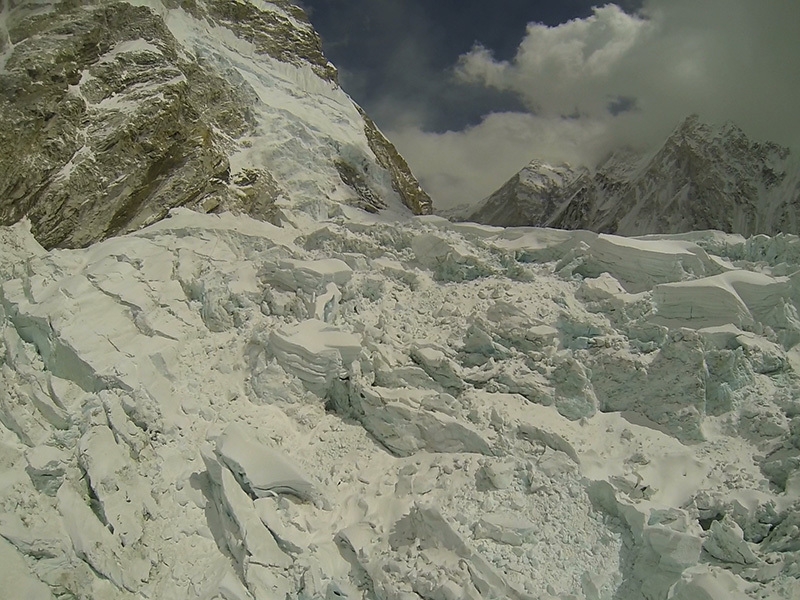In this detailed, up-close photograph, the viewer is transported to the rugged, snowy mountainside near the peak of a remote mountain. The foreground features large, broken chunks of snow and ice, suggesting deep snowpack several feet thick. Just a few feet beyond, a steep, rocky structure emerges from the snow, its jagged surface only partially covered due to its incline. The snow is predominantly white with subtle shading. In the background, additional mountains stretch upward into the sky, their peaks shrouded in fluffy white and gray clouds. The mountainous rocks are gray, contrasting with the surrounding snow. The sky above is a mix of dark blue and white, fluffy clouds, with some areas appearing foreboding under a large gray cloud on the right side of the image. The overall scene captures the serene yet harsh beauty of the high-altitude landscape, revealing hints of paths where people or animals have navigated through the deep snow.